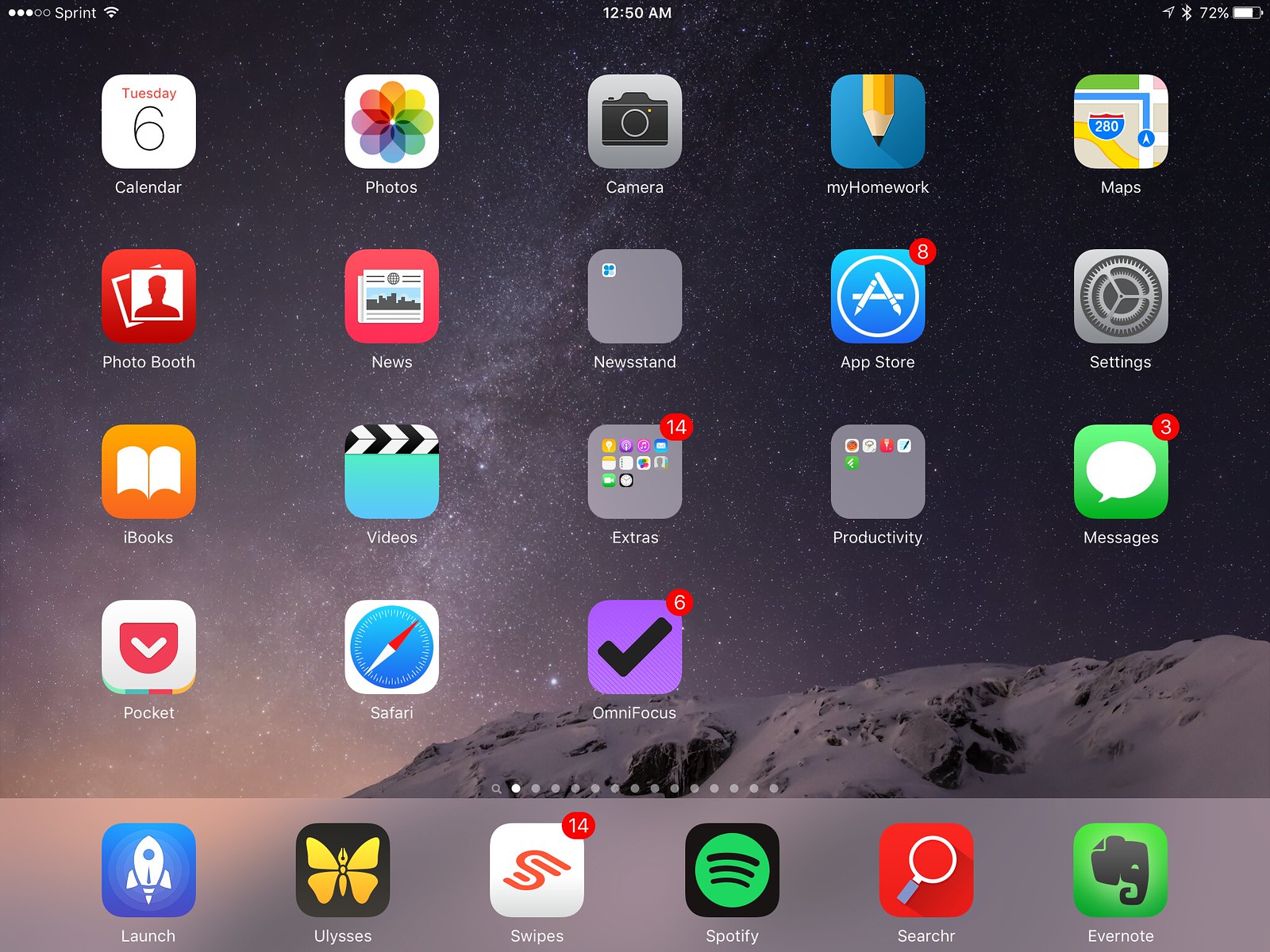A detailed and clean descriptive caption could be:

This screenshot captures the home screen of a smartphone, specifically an iPhone using the Sprint network. At the top of the image, the network signal is depicted with several dots and the word "Sprint," accompanied by a tornado-like symbol indicating Wi-Fi connectivity. The time displayed on the status bar is 12:50 AM. On the right side of the status bar, the battery level is at 72%, and icons for both Bluetooth and location services are active.

The lower portion of the screenshot showcases a row of the device's most frequently used apps, arranged neatly. From left to right, these apps include:
1. A blue square with a white rocket icon labeled "Launch."
2. A black square featuring a yellow butterfly labeled "Ulysses."
3. A white square with a squiggly line labeled "Swipes."
4. The Spotify app icon, which is black with a green circle containing radiating lines.
5. A red square with a magnifying glass labeled "Searcher."
6. A green square with an elephant head representing Evernote.

The background wallpaper of the home screen is an image of a starry purple sky at night, featuring a snow-capped mountain, adding a serene and picturesque touch to the overall visual.